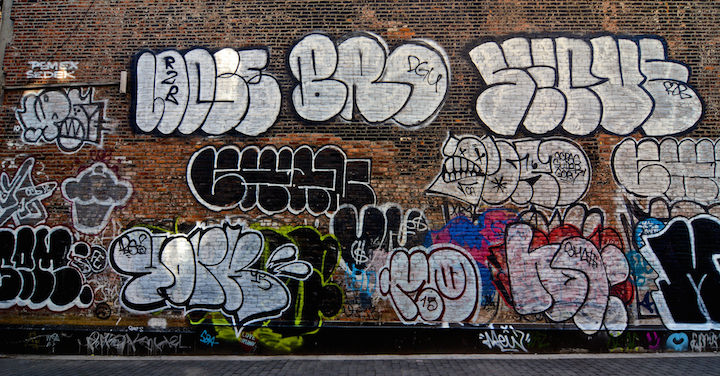This image depicts an old brown and dark brown brick wall, completely covered in vibrant graffiti. The graffiti is composed of large, curvy bubble letters in a variety of colors including red, blue, black, white, grey, green, yellow, and bright pink. Some of the graffiti features intricate lettering that is hard to read, with noticeable words like "bro" and "serve". Among the artwork, specific designs stand out, such as a clenched fist and a cupcake or muffin stencil. The wall is located in an urban setting with a cobblestone street in a gray color visible below. The graffitied wall also showcases several artist signatures, adding to the layering of the street art.